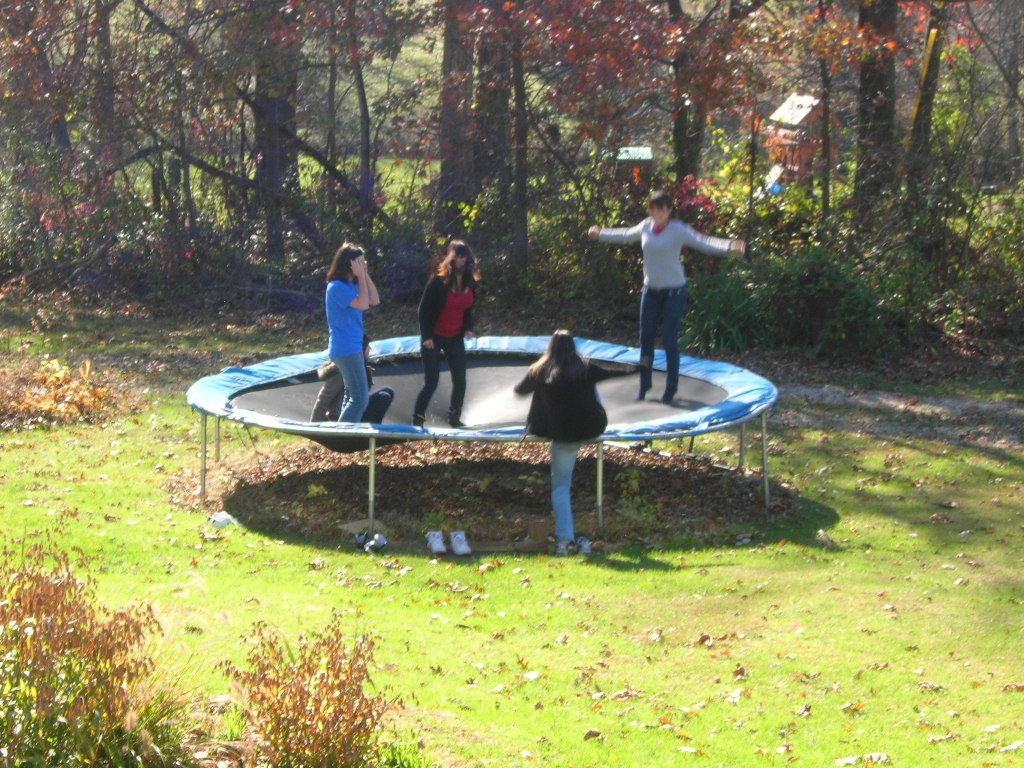A vibrant photograph captures four middle-aged women enjoying a sunny outdoor afternoon in an open yard, surrounded by the brilliant foliage of fall. The yard features lush green grass scattered with dried leaves, and mature trees with a mix of green and orange foliage tower in the background. Dominating the scene is a large, blue-rimmed trampoline with a black surface, centered in the middle of the yard. Three women are energetically jumping on the trampoline: one mid-air with arms splayed out, dressed in black pants and a white shirt; another standing in blue pants and a blue shirt; and the third in a red shirt, black pants, and a black sweater. Nearby, another woman is climbing onto the trampoline in blue pants and a black shirt, and a fourth woman is sitting casually on the edge, dressed in black and gray attire. Around the trampoline, there are multiple pairs of shoes, mostly white sneakers, scattered on the grass and some underneath the trampoline.